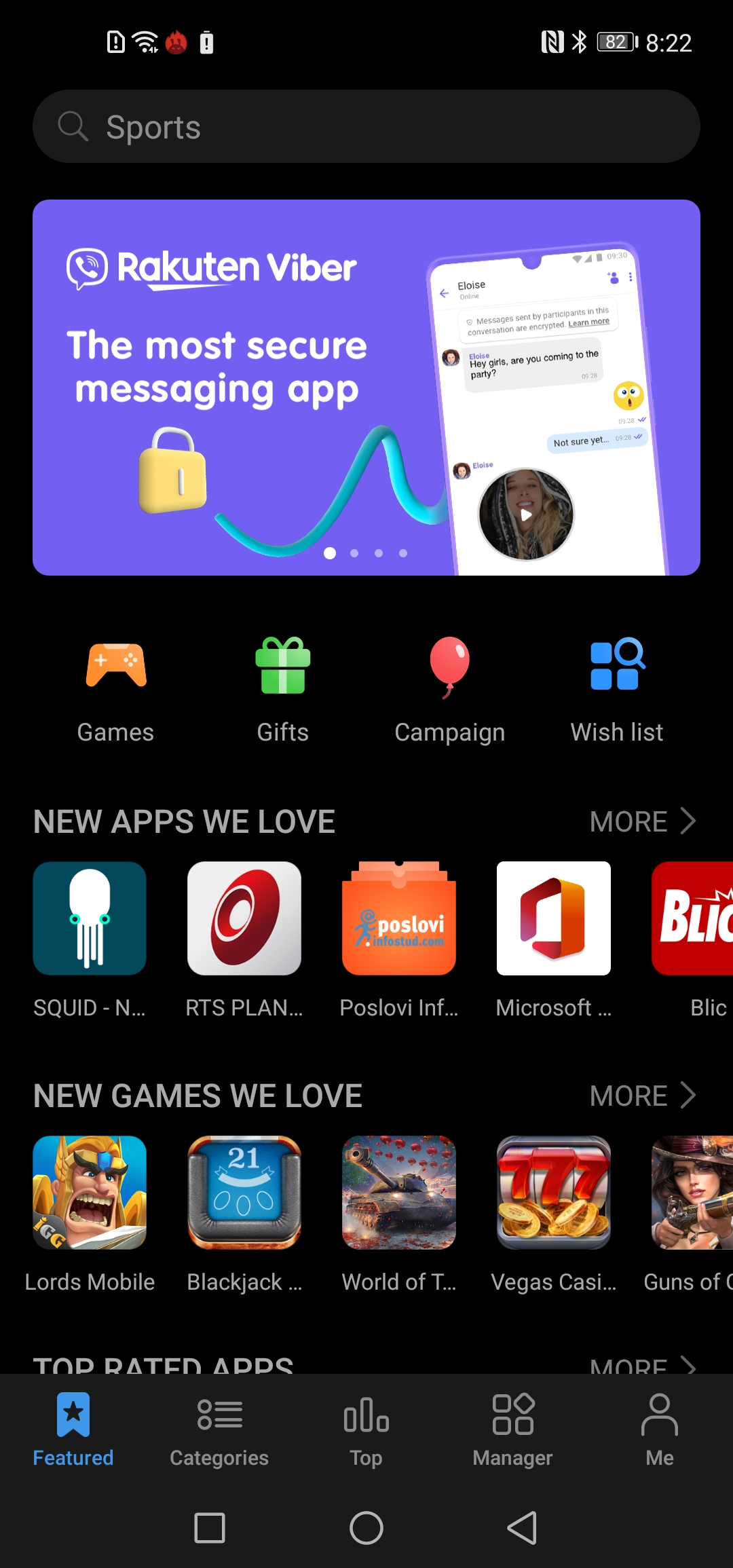The screen in the image depicts an app store interface with a sleek black background. At the top left corner, there are icons representing various phone applications. On the top right, the phone's battery level is displayed at 82%, and the current time is 8:22. 

In the upper section under the app store header, a search bar is prominently featured with a placeholder text indicating "Sports." Directly below the search bar, there is an advertisement banner for "Brockton Viber - The Most Secure Messaging App" which showcases a phone interface displaying a messaging conversation. Next to the phone image is a lock icon, all set against a purple background symbolizing security.

Beneath the advertisement, there are four buttons: "Games," "Gifts," "Campaign," and "Wishlist," each accompanied by an icon that visually represents its function. Following these buttons is a section titled "New Apps We Love," featuring highlighted applications in a carousel format. The apps listed include "Squid," "RTS Plan," "POS Lobby," "Microsoft," and "Blick," each with their respective icons.

Further down, another section labeled "New Games We Love" showcases a selection of games such as "Lords Mobile," "Blackjack," "World of Tanks," "Vegas Casino," and "Guns of [unspecified]." The icons for these games depict various themes such as a warrior, a tank, a woman shooting a gun, and more related imagery.

At the very bottom of the screen, a navigation bar is present with options like "Featured," "Categories," "Top Manager," and "Me," aiding in easy exploration of the app store's content.